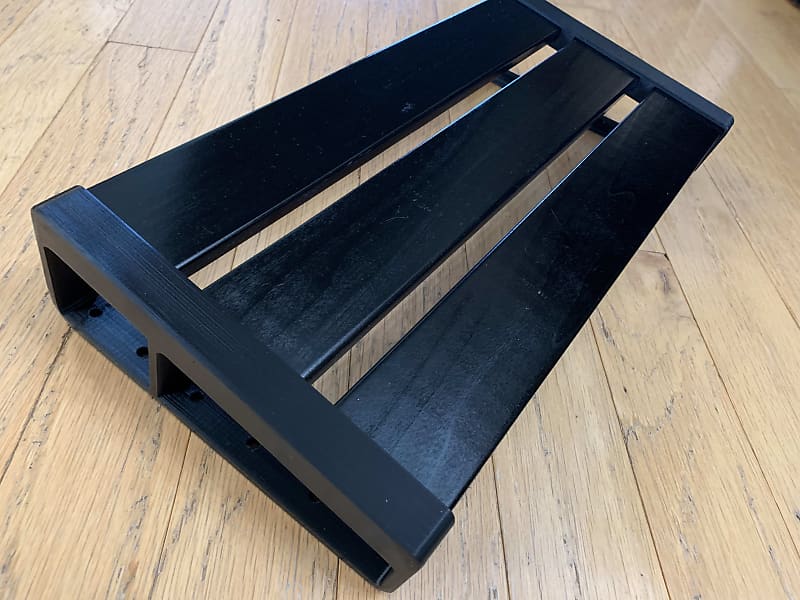The image features an indoor setting with a large, light-colored wooden floor exhibiting some wear and marked details. The floor is glossy and might be made of luxury vinyl, appearing as wood with visible planks and subtle black streaks. Central to the image is a black-painted wooden rack that reveals its wood grain beneath the paint. The rack, resembling a palette or tray, consists of three long, parallel planks with gaps between them, held together by two end caps which are not solid but frame the ends, making the interior visible. The object is somewhat diagonal against the floor, with reflections suggesting possible sunlight.